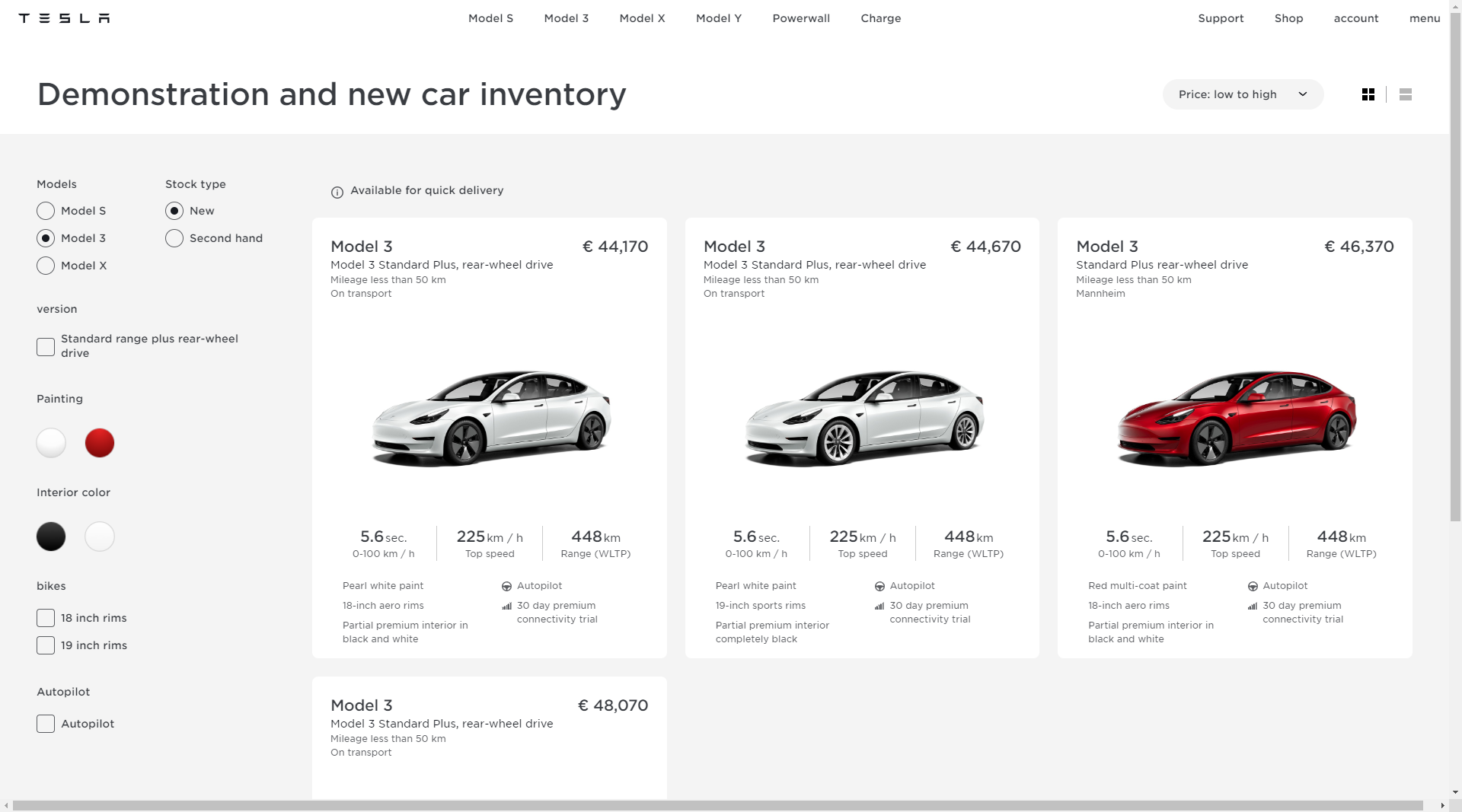This image is a screenshot from the Tesla website with a stark white background. At the top left corner, the Tesla name and logo are prominently displayed. The logo features the "TESLA" name in all capital letters. The "E" is uniquely stylized with three horizontal lines, the "S" has a block-like shape, and the "A" consists of two horizontal lines with extending lines on either side.

Moving across the top menu from left to right, the following categories are listed in gray font: Model S, Model 3, Model X, Model Y, Powerwall, Charging. On the far right, we see the additional options: Support, Shop, Account, and Menu.

On the left side of the page, there is a gray headline that reads "Demonstration and New Car Inventory." Below this headline, the background is a very light gray. A sidebar menu lists the various models again: Model S, Model 3, Model X. It also includes options for "Stock Type" categorized into "New" and "Secondhand." The Model 3 and New options are currently selected.

Within the selection area, options for the Model 3's Standard Range Plus rear-wheel-drive variant are not selected, but details about different paint and interior choices are given. Paint options include white or a dark red, while interior colors include black or white.

The results page showcases three vertical white rectangles, each displaying an image of a Model 3 car. Prices for these cars are listed in euros: €44,170 for one vehicle, €44,670 for another, and €46,370 for the third. Among these models, two are displayed in a very light silver-gray color while the one on the right is presented in dark red.